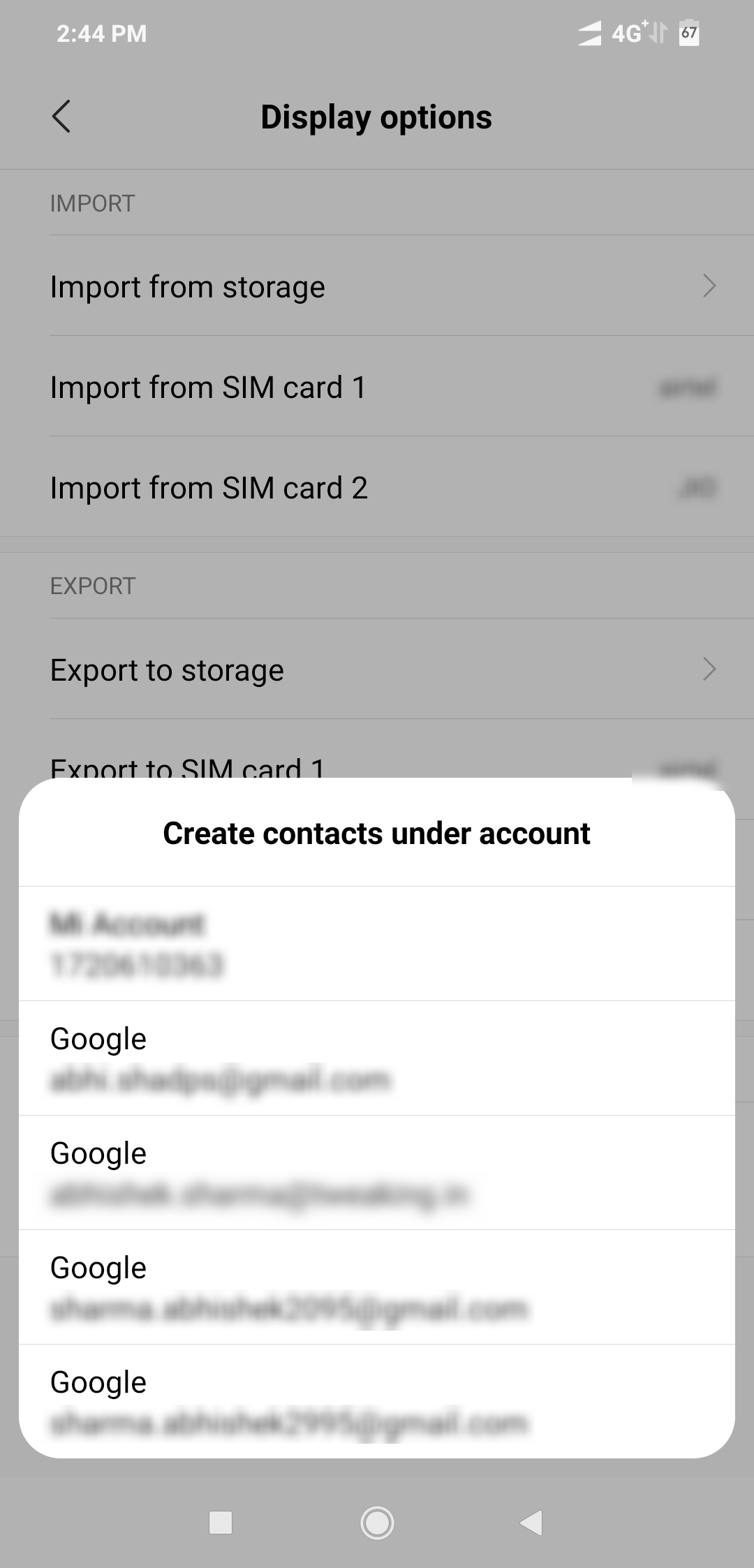This screenshot captures the 'Display Options' section on a mobile phone. The top-left corner shows the current time as 2:44 p.m., while the top-right corner displays the battery level at 67%, and a 4G connectivity icon. This section focuses on display settings for the device.

Directly below this, there are two main sections: 'Import' and 'Export'. The 'Import' section offers three options: 'Import from Storage,' 'Import from SIM card 1,' and 'Import from SIM card 2.' The 'Export' section includes two options: 'Export to Storage' and 'Export to SIM card 1.'

A white pop-up window titled 'Create Contacts under Account' overlaps the lower part of the screen, obscuring additional elements. This window, which features a white background, appears to have had some of its content redacted. It contains five rows, the first of which is fully redacted. The remaining four rows each mention 'Google', but other values are blurred and cannot be discerned.